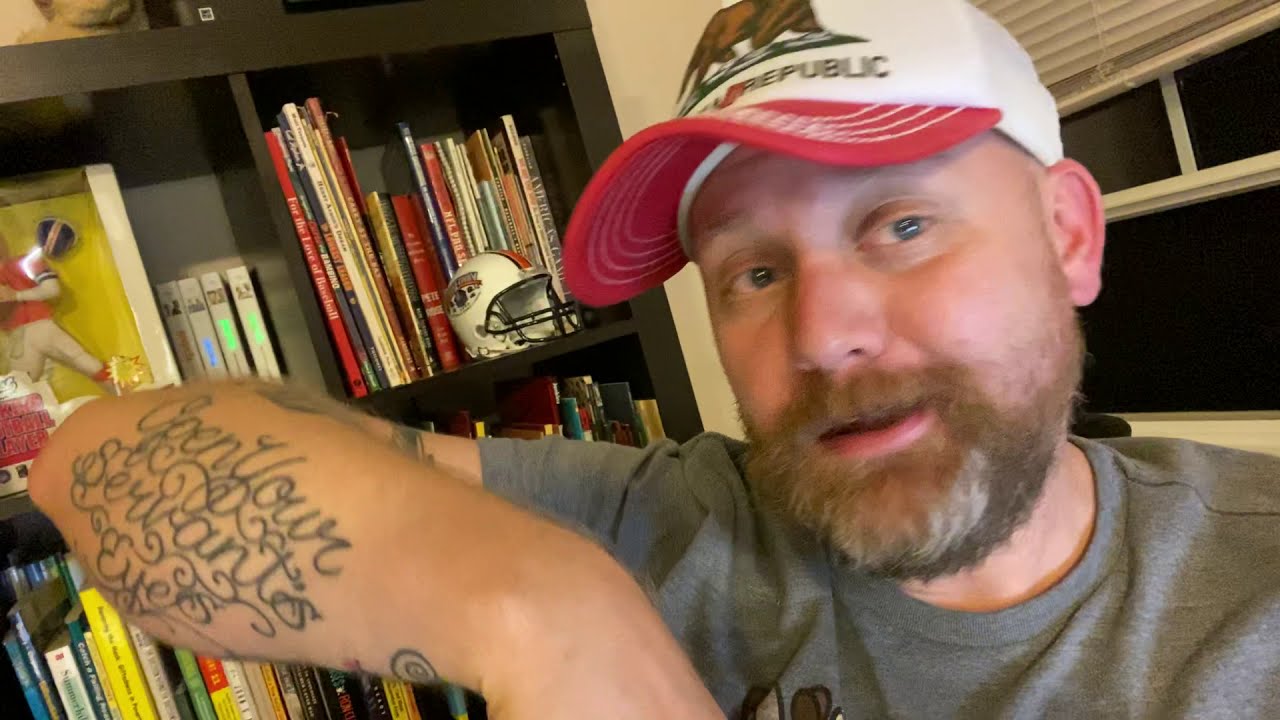This indoor photograph features a Caucasian man in his late 30s to early 40s, seated in front of a dimly lit corner of a room with an open window in the background, revealing a pitch-black night outside. The man has blue eyes and a reddish-brown beard flecked with gray, and he appears to be bald beneath his white ball cap with a red brim featuring a brown bear and the word "Republic." He is wearing a short-sleeved gray shirt and is holding up his right arm to display an intricate tattoo on his forearm. The tattoo, rendered in ornate cursive, reads "Open Your Servant's Eyes" and is surrounded by decorative elements like wires or flowers. Additional tattoos can be seen on the upper part of his arm. Behind him, a black bookshelf holds numerous books and sports memorabilia, including a small white football helmet and a boxed action figure of a football player. The man appears to be speaking, as his mouth is open and his eyes are directed upwards to the right.